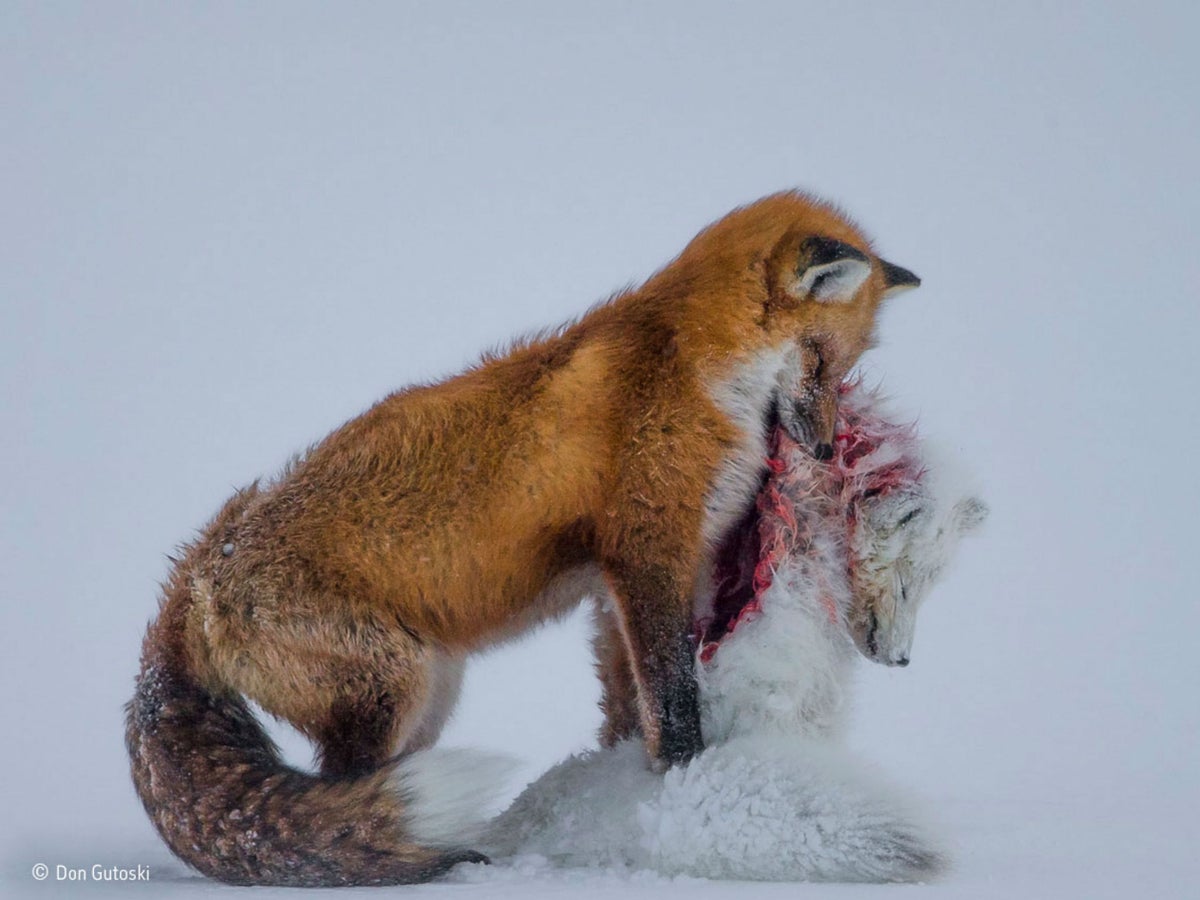A striking red fox is seen holding the lifeless body of a white fox, its mouth gripping the neck or possibly a flap of fur from the deceased animal. The scene unfolds on a snow-covered ground, with the red fox standing slightly elevated by partially positioning its front legs atop the white fox, creating a subtle upward angle. The white fox's head is clearly visible, revealing closed eyes, indicating it is dead. A grisly wound is evident on the back of the white fox, with a red, gaping hole visible just beyond the front leg and chest of the red fox. The red fox has a cream-colored chest, contrasting its vibrant red fur, with black-tipped ears and darker markings around its legs and tail. The fox's grimacing expression, with tightly closed eyes and perked ears, adds to the dramatic intensity of the moment.